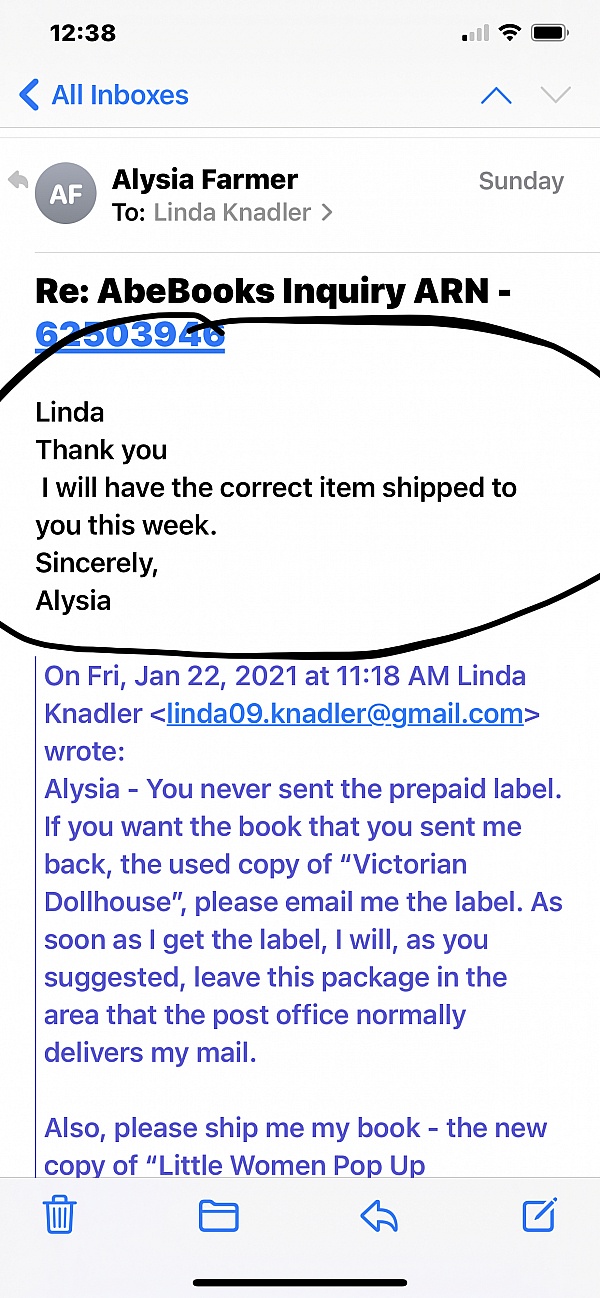This image seems to be a snapshot of a smartphone screen showing an email or messaging application. At the top of the screen, the time reads 12:38, and to its right is a signal strength icon displaying four bars, with only one bar filled. Next to the signal bar, the Wi-Fi icon is fully filled, indicating a strong connection. Further to the right, a fully charged battery icon is visible.

Below this status bar, a grey banner displays. On the left side of this banner, there's a blue left-pointing arrow, and next to it, the text "All Boxes" is highlighted in blue. To the right side of this banner, there are two arrows; a blue one pointing upwards, and a light grey one pointing downwards.

Underneath the banner, there is a small white space followed by the name "Alicia Farmer." On the left, there's a grey circle with the initials 'AF', and to the right, the text "2" followed by "Linda KNADLER" with a right-facing arrow. The word "Sunday" is displayed at the top right.

The main body of the message begins with the text "Read Add Books Inquiry ARN," which seems to be highlighted with a black circle. Below that, the text from Alicia reads: 

"Linda,
Thank you. I will have the correct item shipped to you this week.
Sincerely,
Alicia."

Further down, additional information such as the date, the name "KNADLER," a Gmail address, and previous communication from Alicia and the term "dollhouse" are seen, leading into another partially visible paragraph.

At the bottom of the screen, some icons are visible but not clearly defined.

This detailed depiction of a screen capture offers a comprehensive view of the interface and the message content.